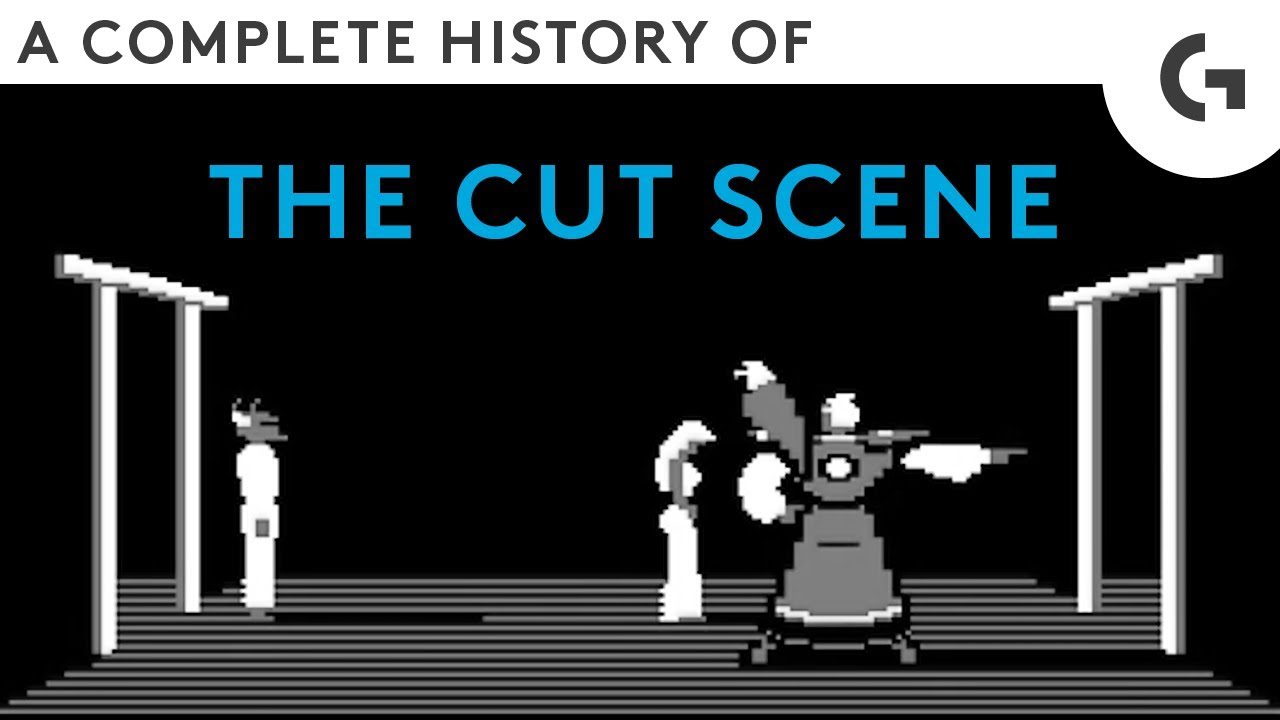The image is a digitally styled poster titled "A Complete History of the Cut Scene" with the words "the cut scene" prominently displayed in blue block letters within a black box. The scene is pixelated, reminiscent of video game graphics, and shows three characters standing on a patterned black and white floor. On the left, there is a figure that appears to be a man or possibly a demon wearing a white karate outfit with a black belt. In the middle, a woman with blonde hair, dressed in a two-piece white outfit with her head bowed and looking to the right, stands next to a wizard-like character. This wizard figure is dressed in a long robe with outstretched arms, one of which is pointing and creating a puff of smoke or magical effect. The setting is framed by two large white archways or gates on each side, contributing to the dramatic and somewhat mystical ambiance of the scene.